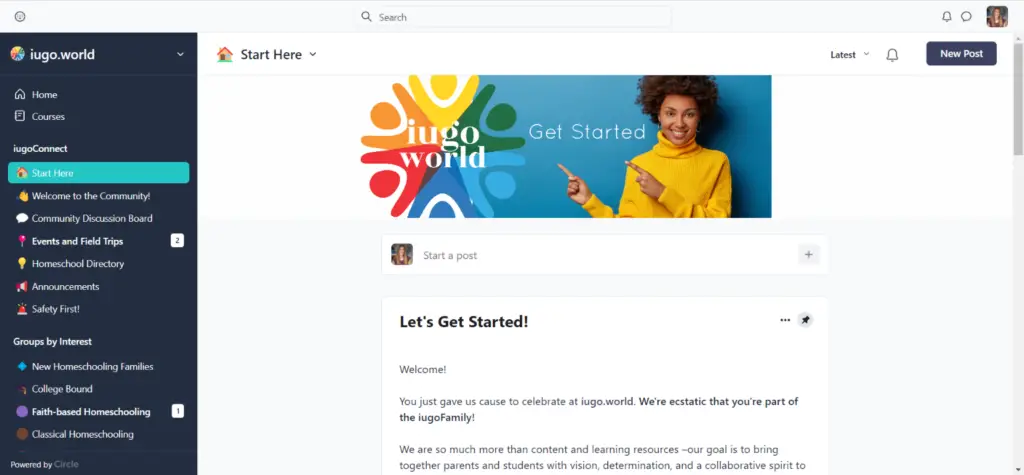The image displays the IUGO.world website with a vertical navigation menu on the left-hand side. At the top of the menu is the label "IUGO.world" accompanied by a drop-down arrow. The menu is organized into multiple sections:

1. **Home**
2. **Courses**
3. **IUGO Connect:**
   - Start Here
   - Welcome to the Community
   - Community Discussion Board
   - Events and Vale Trips
   - Homeschool Directory
   - Announcements
   - Safety First

4. **Groups by Interest:**
   - New Homeschooling Families
   - College-Bound
   - Faith-Based Homeschooling
   - Classical Homeschooling

To the right side of the screen, occupying the main window of the website, is a "Let's Get Started" section featuring a person pointing towards the "IUGO.world" emblem. The layout and design of the website appear to be user-friendly, catering to various aspects of homeschooling and community engagement.